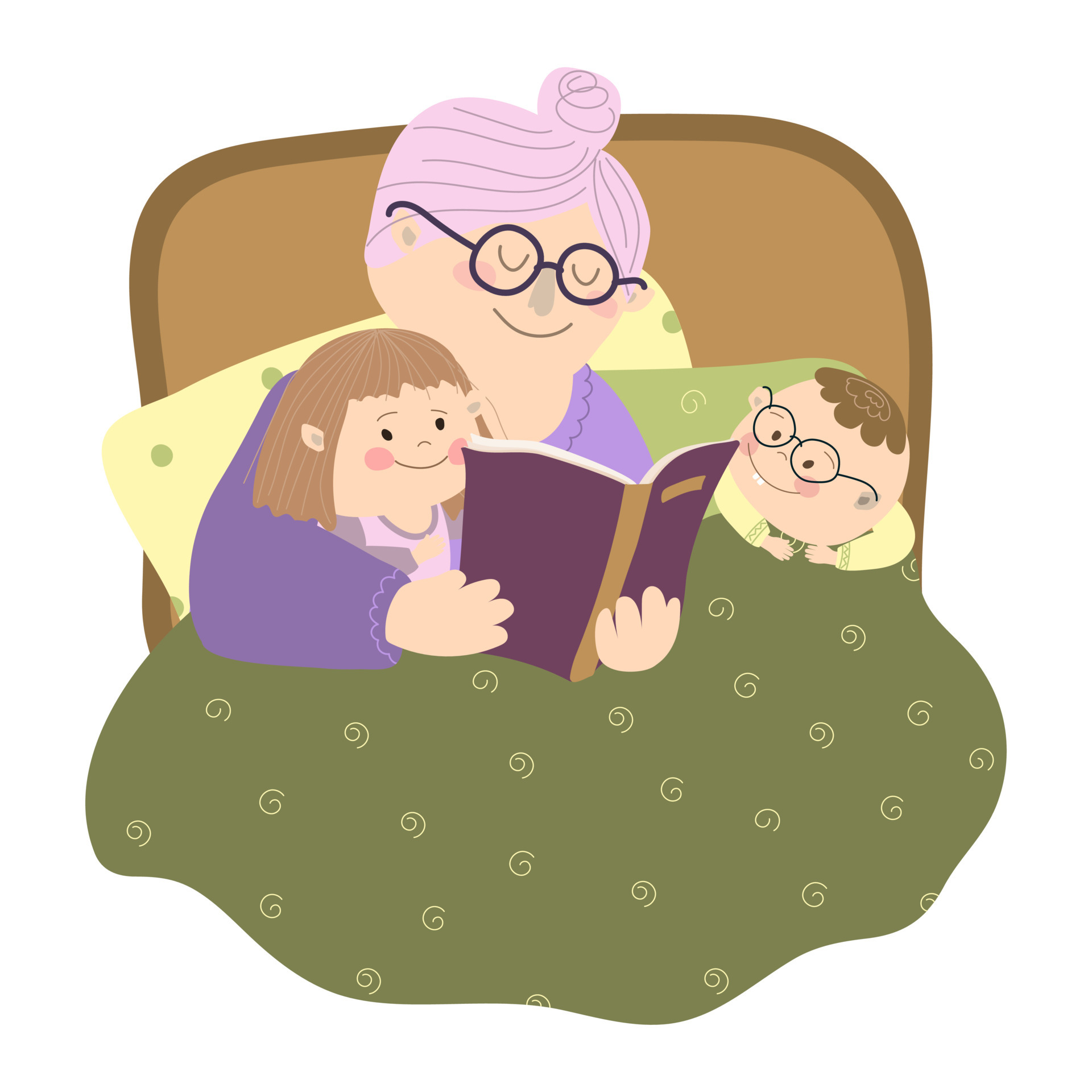In this vibrant cartoon-style illustration, a grandmotherly figure with a tight, light purple bun is lovingly reading a purple book with a brown binding to her two grandchildren while nestled together in a bed. The grandma, who is wearing round black spectacles and a cheerful smile, dons a purple nightgown and leans against a green pillow adorned with darker green polka dots. Her eyes gently closed, she delights in sharing the story. Her granddaughter, positioned to the left, mirrors her joy with a broad smile, rosy cheeks, and a short brown bob. She is cozy in a pink and purple nightgown. To the right, the grandson, a toddler with short brown hair, also wears round glasses and beams with excitement. Clad in a yellow long-sleeve shirt, he leans against a slightly darker green pillow with a swirl pattern. All three share the warmth of an olive-green blanket, also featuring the swirl design, wrapped snugly around them. The setting is completed by a bed with a beige headboard with brown trim, enveloping the happy family moment.